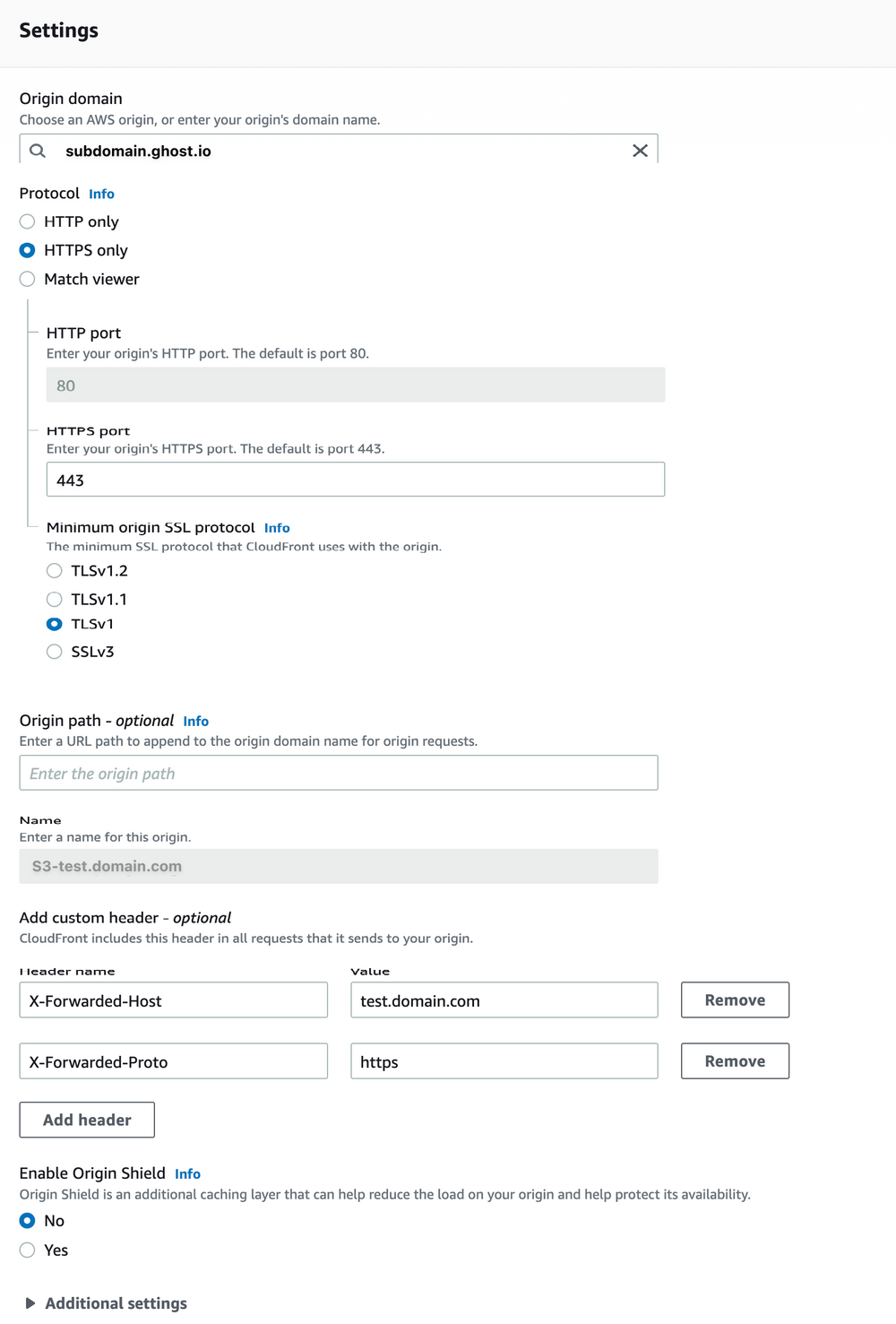**Detailed Description of a Settings Page Image:**

The image showcases a settings page displayed on a minimalist white and gray background. Prominently positioned in the upper left-hand corner, the word "Settings" is written in bold, black font.

Directly below this heading is the section labeled "Origin Domain". This section prompts the user to either choose an AWS origin or manually enter a domain name. An example provided is "subdomain.ghost.io".

Further down, the "Protocol" section appears with options to specify the desired protocol type, including "HTTP Only", "HTTPS Only", and "Match Viewer". The option "HTTPS Only" is highlighted with a blue dot, indicating it is currently selected.

Following the protocol options, users are instructed to enter ports for HTTP and HTTPS traffic. The default HTTP port, labeled "HTTP Port", is set to 80. Similarly, the default "HTTPS Port" is listed as 443.

The "Minimum Origin SSL Protocol" section specifies the lowest SSL protocol that CloudFront will use with the origin. The option "TLSv1" is selected, marked by a blue dot.

An "Origin Path" section is provided as well, labeled optional. This allows the user to append a URL path to the origin domain name for origin requests.

Under "Origin Path Name", users are prompted to enter a name for the origin. An example provided is "S3testdomain.com".

An optional section titled "Add Custom Header" allows CloudFront to include custom headers in all requests it sends to the origin. This part features fields for header name and value, accompanied by remove buttons for each header.

Finally, the "Enable Origin Shield" option is detailed, explaining that enabling Origin Shield adds an additional caching layer to help reduce the load on the origin and protect availability. The options are simply "Yes" or "No", with "No" currently selected.

This settings page provides a comprehensive and organized interface for configuring various aspects of an AWS origin domain, ensuring flexibility and security for the user.